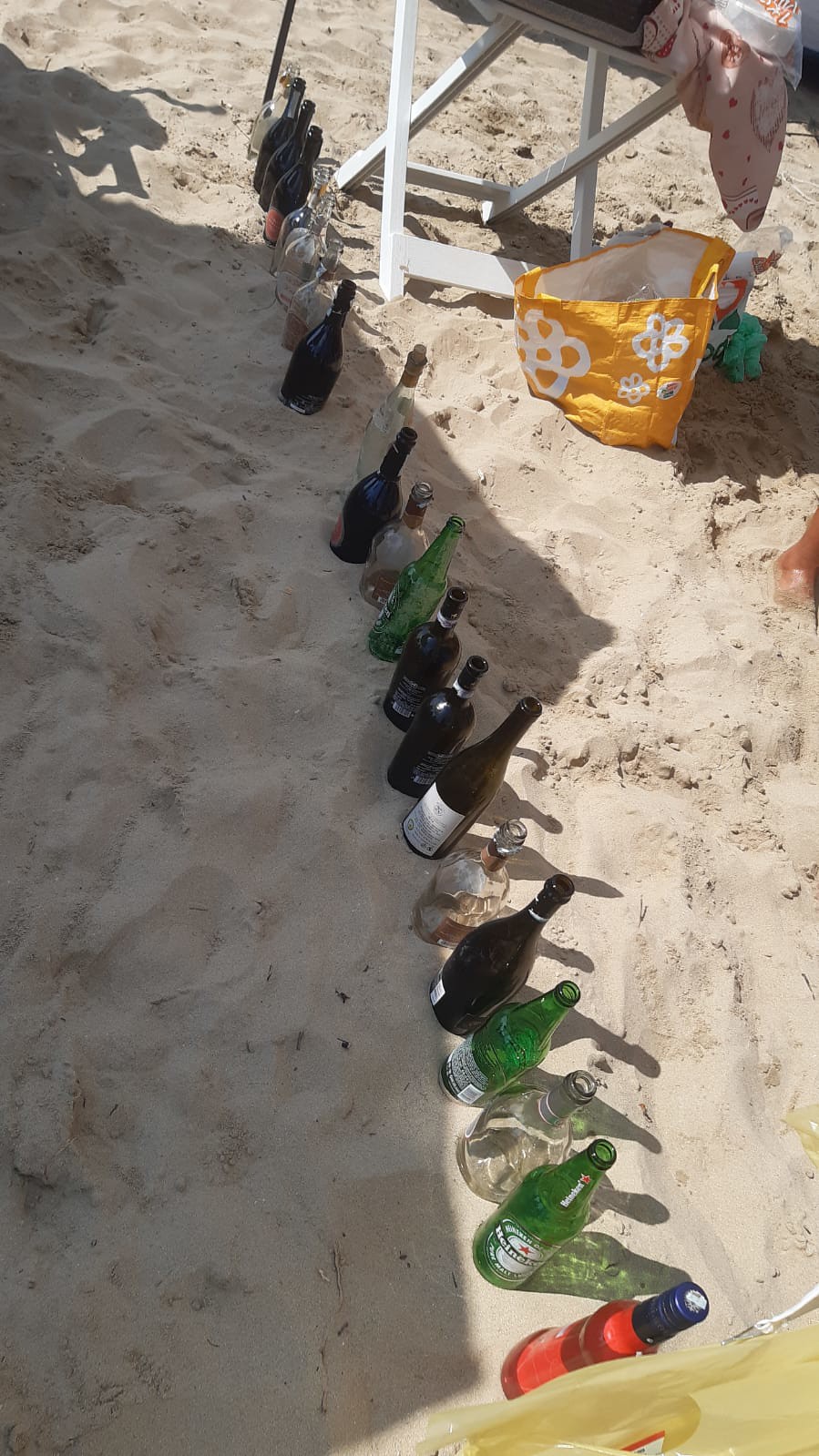The photograph captures a sunny day at the beach, showcasing a scene filled with aftermath festivities. Dominating the image is a straight line of 18 empty alcohol bottles—ranging from wine to beer and spirits—organized in a row on the pale beige sand. The bottles are of various types and colors, including clear, brown, and green, creating a colorful display of the gathering. To the right of this orderly chaos, there's a white folding beach chair adorned with a pink top or sweater draped over it, decorated with dark pink dots. Beside the chair, a gold beach bag with a white floral design adds a splash of color and functionality. Shadows cast over half the photo hint at the bright, sunlit day that preceded this moment. The image, framed mostly at ground level, subtly includes various footprints in the sand, adding depth and a sense of activity. Overall, it’s a vividly detailed snapshot of a beach bash, documenting both the festive lineup of empty bottles and the casual beach setup.